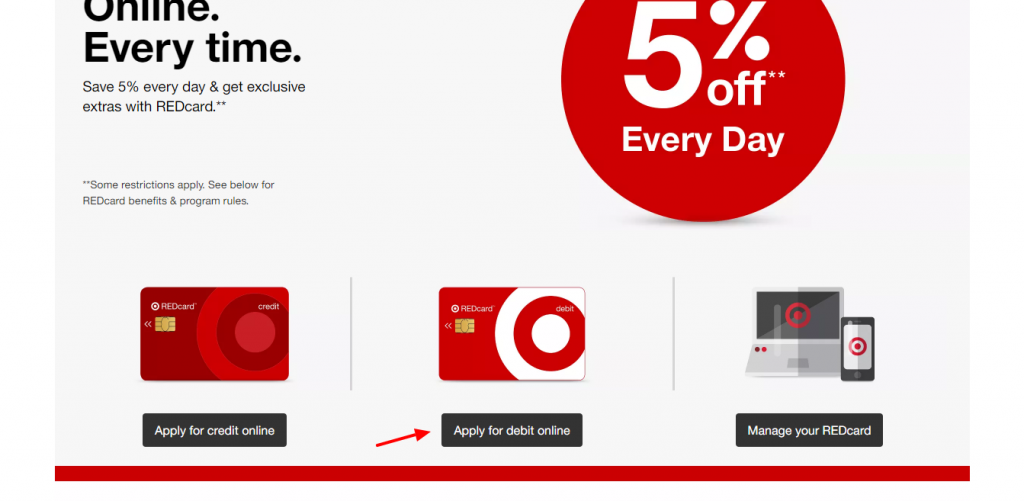Screenshot of Target's Credit Card Advertisement

This screenshot captures an advertisement for Target-branded credit cards featured on Target's website. Dominating the top right corner, a prominent red circle with white text advertises a "5% off every day" discount for using the Target REDcard. The page promotes several financial products: the Target Credit Card, the Target Debit Card, and the option to manage the REDcard, which is the name of Target's exclusive credit card. 

In the center of the image, three horizontally listed links allow users to either "Apply for Credit Online," "Apply for Debit Online," or "Manage Your REDcard." Each link is accompanied by a small icon – either a credit card or a computer – indicating the respective action.

The top left of the image features black text stating, "Online Every Time, Save 5% Every Day, and Get Exclusive Extras with REDcard," summarizing the benefits of the card. The overall layout has a clean, white background, except for a horizontal red bar at the very bottom, reinforcing Target's brand identity. This advertisement highlights the convenience and savings offered by Target's REDcard.